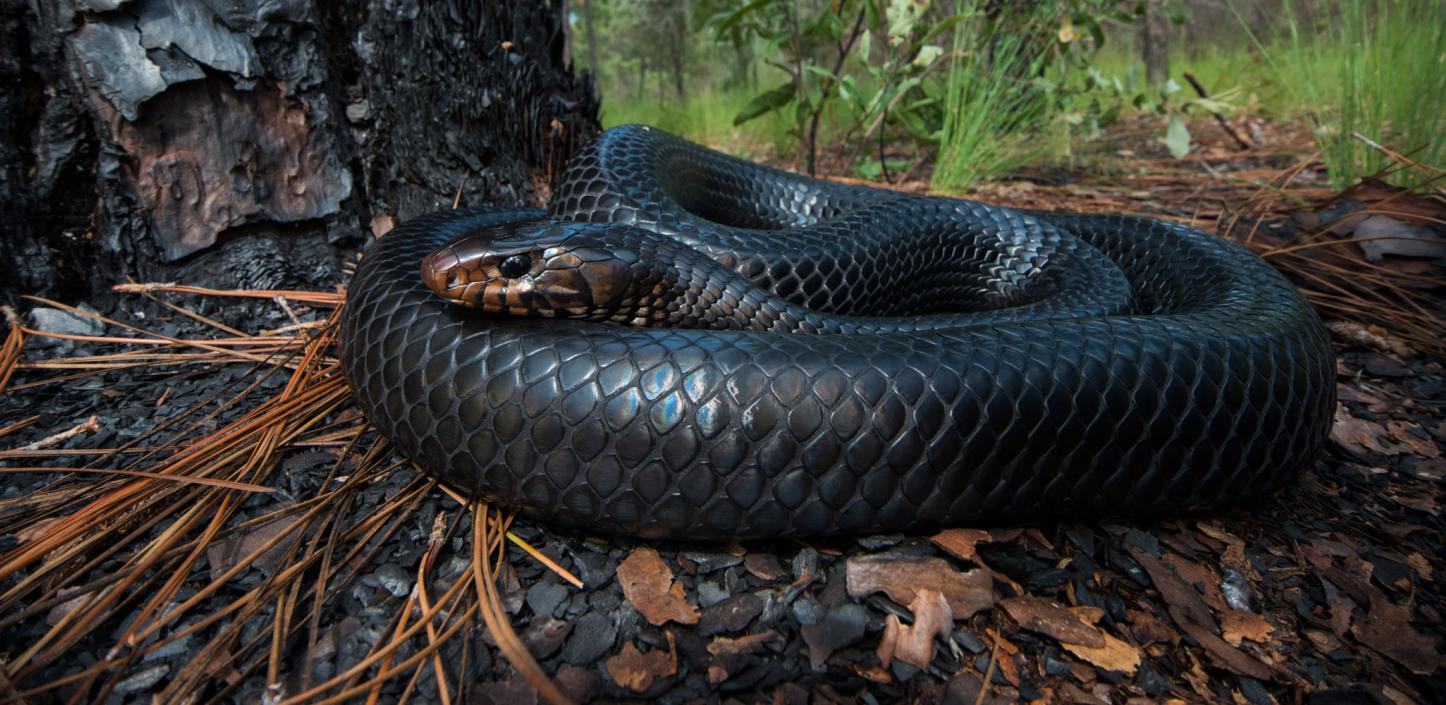In this landscape-oriented close-up photo, a large, predominantly black snake is depicted curled up on a forest floor. The snake's body, which glistens with a glossy sheen, is mostly black, with a hint of brassy, bronze coloration near its nose and mouth area extending to its neck. Its black, textured scales feature subtle diamond-shaped patterns. The snake is positioned near the base of a dark tree trunk, nestled among dried pine needles, brown chunks of bark, and other forest debris. In the background, a mix of trees and grassy terrain can be seen, adding to the natural, outdoor setting. The snake's head rests on the left side of its coiled body, its rounded nose and very black eyes clearly visible, suggesting it isn't a viper.